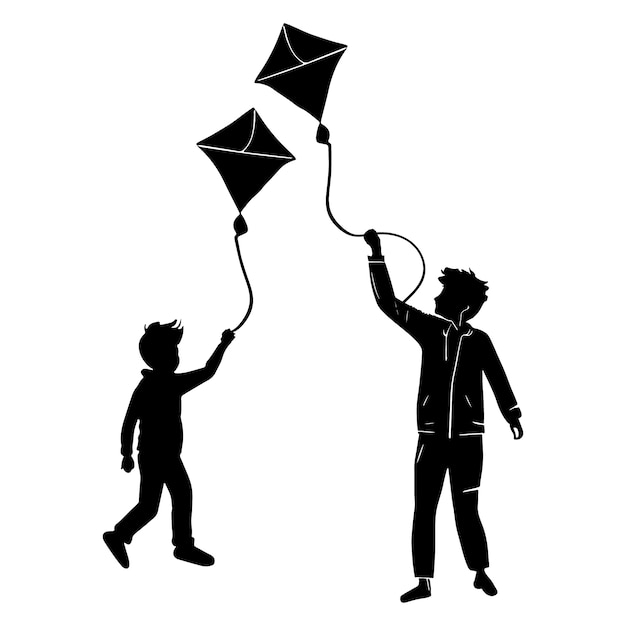In a black and white, clip art-style digital illustration, two figures are depicted flying kites against a stark white background. On the right stands a taller figure, facing the viewer. This person is attired in pants and a jacket, with their right hand raised skyward, grasping a string attached to a high-flying, diamond-shaped kite. The kite’s design features a solid triangle at the bottom and two smaller triangles at the top, with some white lines through the center and a drooping line connecting the kite's segments. 

To the left, a much shorter figure—suggestively a younger child with feathery, wispy hair—also reaches up with their right hand to hold the string of their own lower-flying kite. This child is dressed in long pants, shoes, and a long-sleeved shirt. Both figures are almost entirely silhouetted in black, with minimal white detailing providing contrast. Below each kite, there’s a vague, amorphous circle, adding to the composition's simple yet evocative aesthetic.